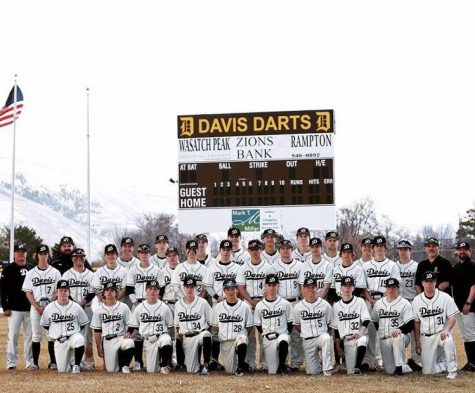This is a detailed photograph of a high school baseball team posing for a team photo at their field. The team members, wearing white uniforms with their team name and numbers on the chest, are arranged in three rows: the first row is kneeling with ten players, the second and third rows are standing. On the left end of the first row stands a coach in a dark top and white pants, while two other coaches in dark shirts stand on the right end. Behind the team, the brown and white scoreboard proudly displays "Davis Darts" at the top in gold letters flanked by two ornate Ds. Beneath are advertisements for Wasatch Peak, Zions Bank, and Rampton. The scoreboard includes sections for Guest, Home, At Bat, Ball, Strike, and Out. Visible in the distant background are a line of trees, a pole with an American flag to the left, and a backdrop of sunlit hills or possibly snowy mountains, with some yellowed grass in the foreground, suggesting the photo was taken in early spring or late fall.